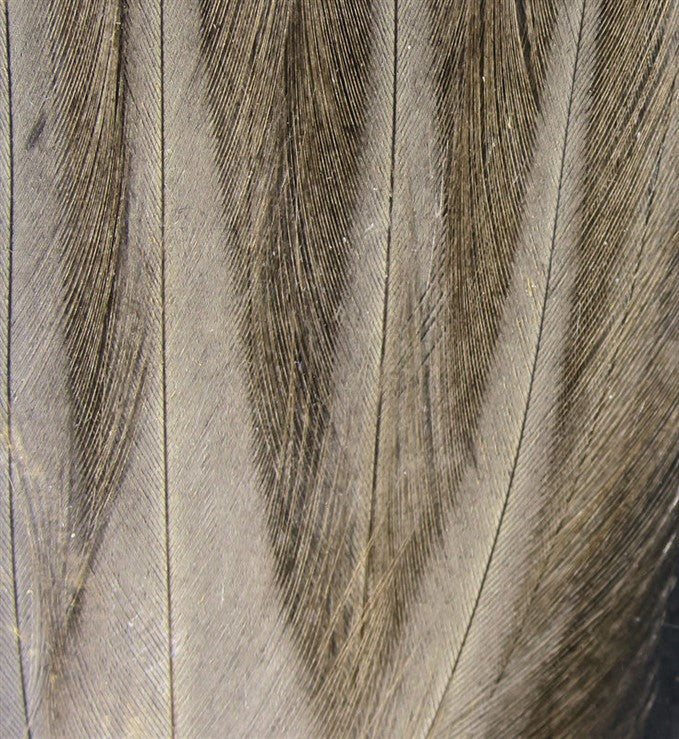This is a detailed, close-up photograph of an intricate wooden texture that remarkably resembles a cluster of feathers. The image is so zoomed-in that the true nature is obscured, but the textures and patterns strongly suggest feather-like structures. These structures exhibit various overlapping fibers, giving a concave appearance and a sense of depth. The lines and patterns are detailed, with color variations that range from shades of brown and tan to light brown and beige, and even some gray. The lighter background might consist of similarly feather-like textures, adding to the complexity and visual interest of the image. The grain of the texture sweeps inward from the sides, converging towards the center, which enhances the feather-like design. Overall, the photograph presents a rich tapestry of hues and intricate patterns that evoke the delicate structure of feathers.